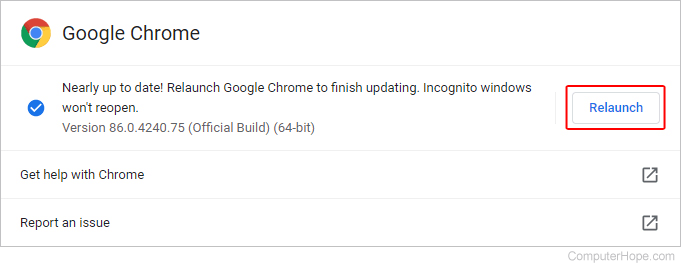The image is a horizontally rectangular frame outlined with a thin light gray border. Just outside this border, at the bottom right, the text "ComputerHope.com" is displayed in light gray. Within the frame, the upper left corner features the Google Chrome icon accompanied by the text "Google Chrome." Below this, a blue checkmark icon is followed by the message "Nearly up to date. Relaunch Google Chrome to finish updating. Incognito windows won't reopen." The text continues with "Version 8.6.0.4240.75" (specified as the official build and 64-bit). On the far right side of this notice, there is a red-outlined "Relaunch" button. Returning to the left side, below the main update message, there are two options: "Get help with Chrome" and "Report an issue."